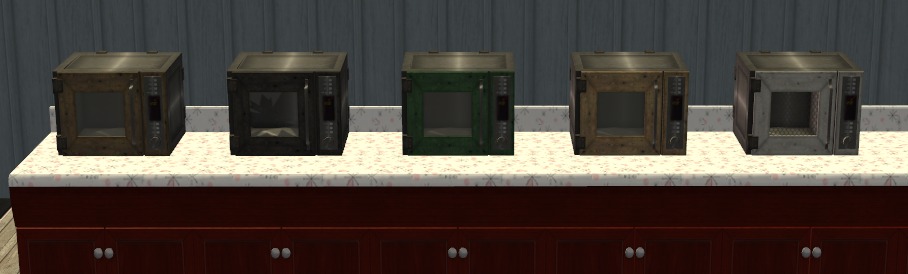The image is a realistic, color photo, likely captured in a display room. It features a spacious, digital recreation of a 3D-rendered cabinetry scene. The long, dark brown base cabinet sports a series of double doors—five sets can be counted, but the cabinetry extends further right, suggesting additional sets. The countertop, spanning from the left side and extending off the right, is made of white marble with goldish marbling, creating a sophisticated contrast against the cabinet. A low backsplash rises a few inches at the back.

Sitting atop the counter are five identical metal devices, differing only in the color of their doors. These colors include gold, gray, green, yellow, and white, while their tops remain uniformly silver with identical reflections. The devices feature a square door on the left side and a rectangular section on the right that includes what appears to be a knob at the bottom. Despite some confusion about their purpose—mini microwaves, safes, or perhaps jewelry boxes—their design suggests a display intent, adding a modern touch to the space with their metallic finishes. The backdrop includes a blue paneled wall, complementing the tan paneled floor below, completing the elegant and polished aesthetic of the room.